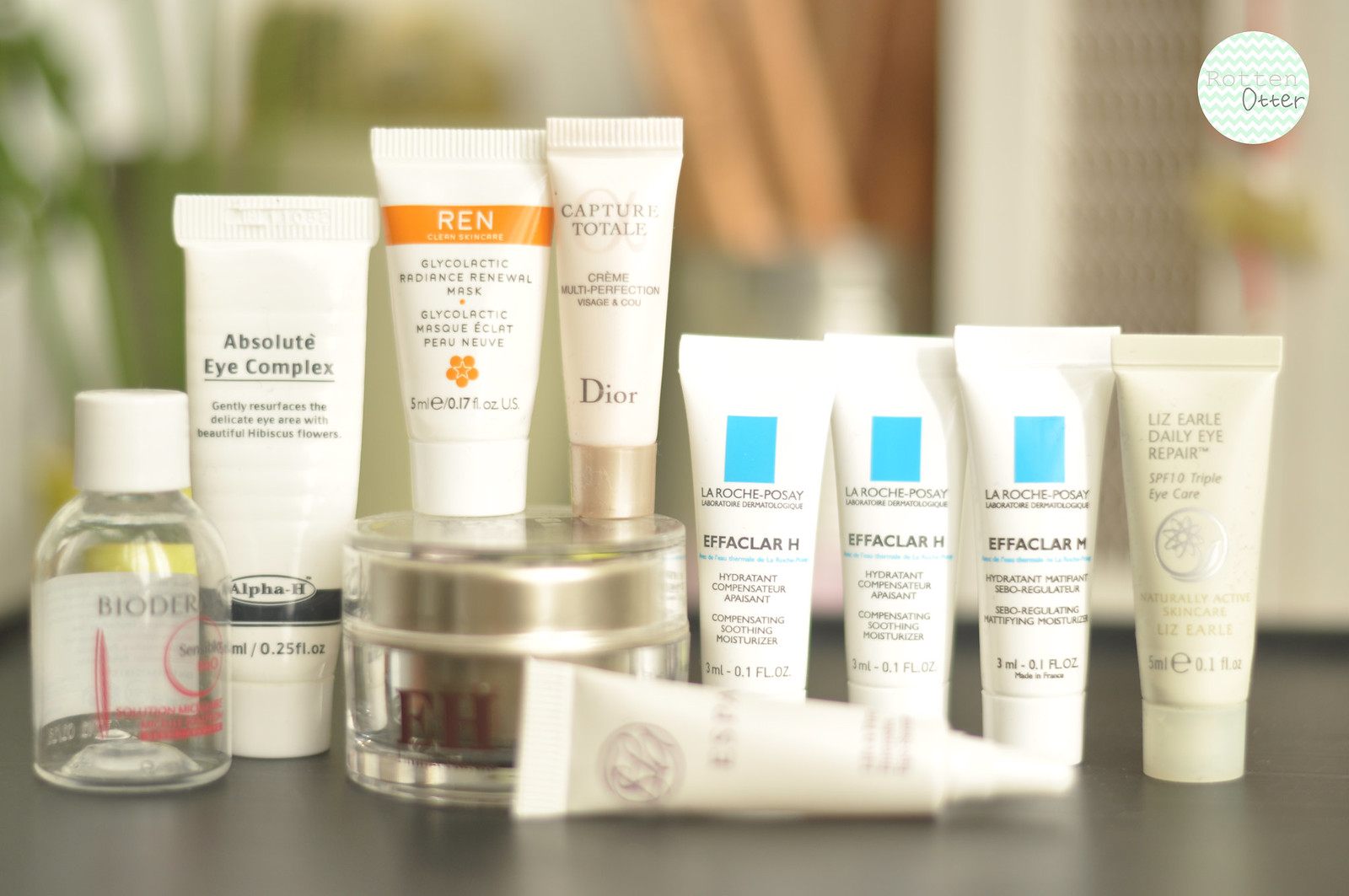This meticulously arranged photograph showcases a diverse selection of skincare products, neatly aligned against a minimalist backdrop. Starting from the left, the lineup begins with a small clear bottle featuring a white cap, possibly branded with the name "Bioderb" in black lettering, though the text is slightly blurred. Adjacent to it, a white tube stands upright with its cap positioned at the bottom; this is labeled "Absolute Eye Complex" from Alpha-H, containing 0.25 fluid ounces of product.

Next in line is a round, clear container, about an inch in height, carrying visible "EH" initials. Resting on top of this is another white tube with a bottom cap; this one displays the "REN" brand in white letters set against an orange background, and it is identified as a "Glycolactic Radiance Renewal Mask" containing 0.17 fluid ounces.

Further to the right is a white tube from Dior, marked "Capture Totale," a multi-perfection face cream distinguished by its bronze cap. Beside it, three identical white tubes, emblazoned with "La Roche-Posay Effaclar H," each hold 0.1 fluid ounces and feature the brand’s signature blue rectangle.

Continuing rightward, there's a beige tube labeled "Liz Earle Daily Eye Repair SPF 10 Triple Eye Care," also containing 0.1 fluid ounces. Lying in front of all these products in the foreground is another out-of-focus tube, adding depth to the composition.

In the top corner of the image, a photoshopped logo reads "Rotten Otter," encircled by a pattern of green zigzags, adding a touch of branding to the scene. The overall effect is a polished and detailed display of varied skincare essentials, artfully presented to capture the attention of the discerning viewer.